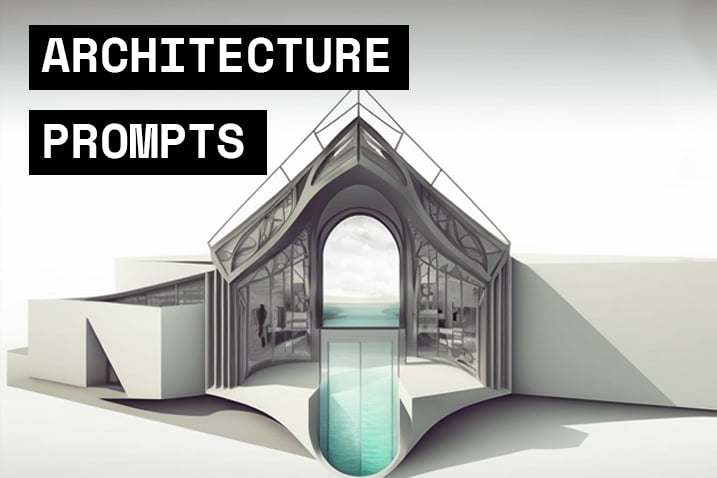The image depicts a highly detailed 3D architectural rendering in landscape orientation. The primary subject is a minimalist yet intricate building, set on an oceanfront. The building features white stucco walls on both the right and left sides, and its central section showcases an elaborate gable roof structure made of gray steel. Beneath this roof is an arched opening that provides a panoramic view of the shimmering aqua ocean in the distance. This opening also includes a see-through glass panel at the base, allowing a view of the seawater below. White walkways flank this central section on either side. The entire scene is bathed in a blend of light colors, primarily a palette of light blue-green, gray, white, and black. The background gradient shifts from darker at the top to lighter in the middle, and then slightly darker again at the bottom. In the top left corner, white text reading "Architecture Prompts" is enclosed in two black horizontal rectangles, rendered in a custom serif font. This image likely represents a screenshot from a presentation or online instructional video, emphasizing the sleek and modern design elements of the architectural concept.